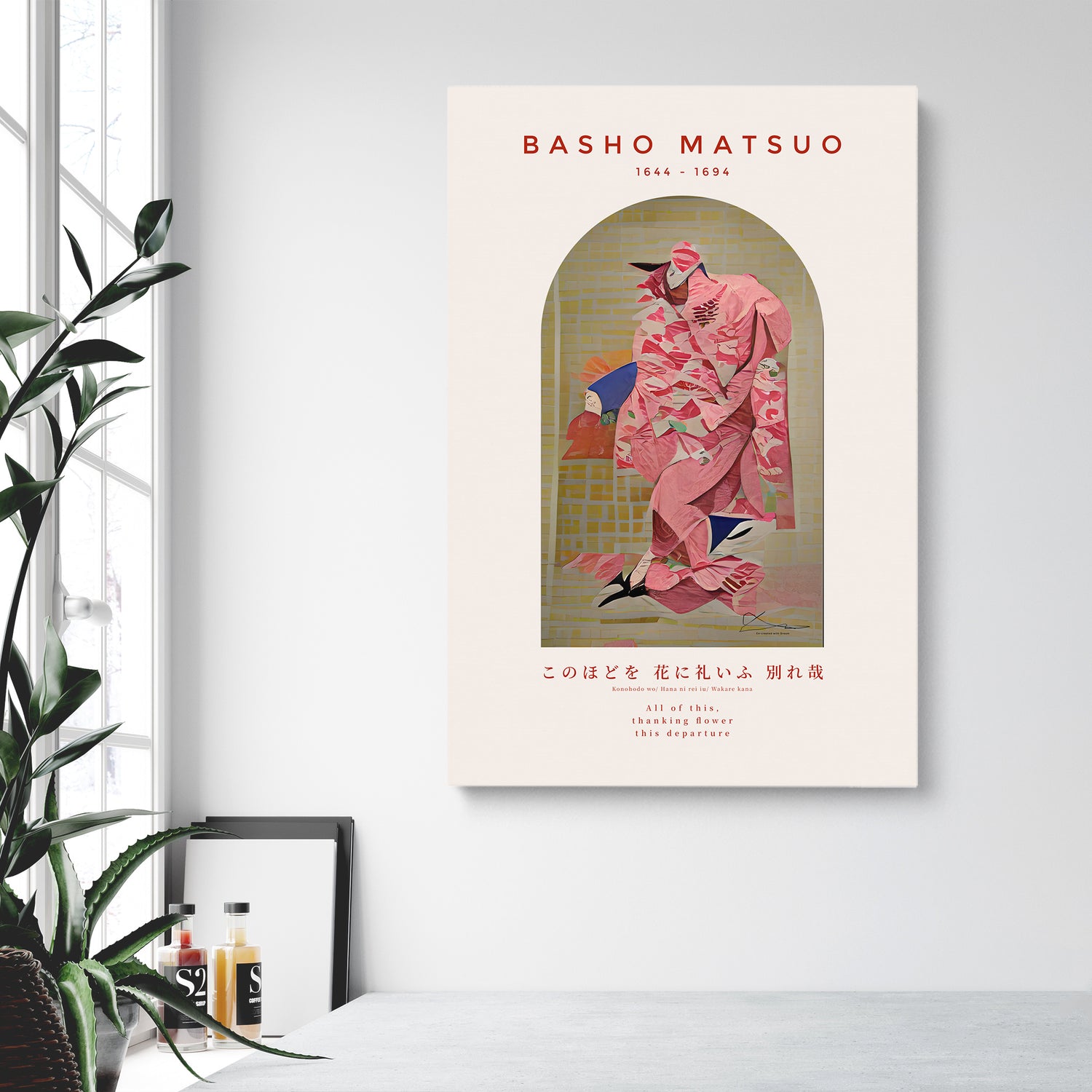In the corner of the room, there is a serene setting featuring a white wall and a white window to the left. On the windowsill sits an aloe vera plant alongside some tall green plants, creating a touch of nature indoors. The white wall hosts a visually striking poster titled "Basho Matsuo, 1644-1694," featuring a drawing of a human figure adorned in a long pink robe, possibly a kimono, against a cream-colored background with a subtle green hue. Below the title are Japanese characters that add an authentic touch to the poster. At the corner where the window meets the wall, two bottles of liquid stand side by side—one red bottle on the left and one yellow bottle on the right, adding a subtle splash of color to the composition.